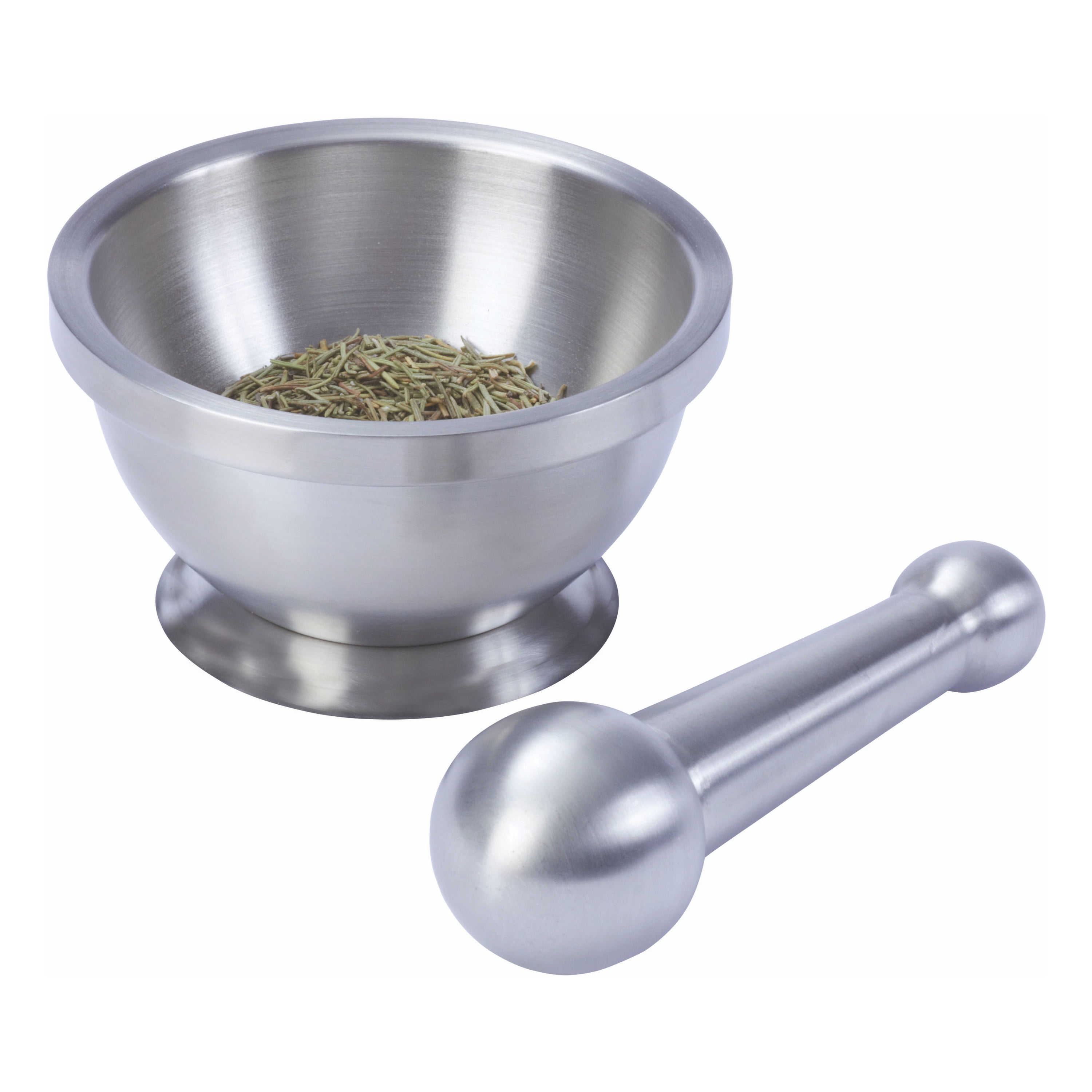This photograph features a white background highlighting a shiny, silver-colored metal mortar and pestle in the foreground. The focal point is a small, cylindrical metal bowl, resembling a material such as aluminum or steel, containing green herbs that appear to be rosemary, based on their thin, needle-like leaves. Resting horizontally outside the bowl is the pestle, distinguished by its cylindrical shape with two knobs on either end, the larger knob presumably designed for effective grinding. This setup, typically ceramic in construct, presents a unique modern twist with its sleek, steel-like appearance, suggesting the herbs are ready to be ground down into powder for culinary or medicinal use.